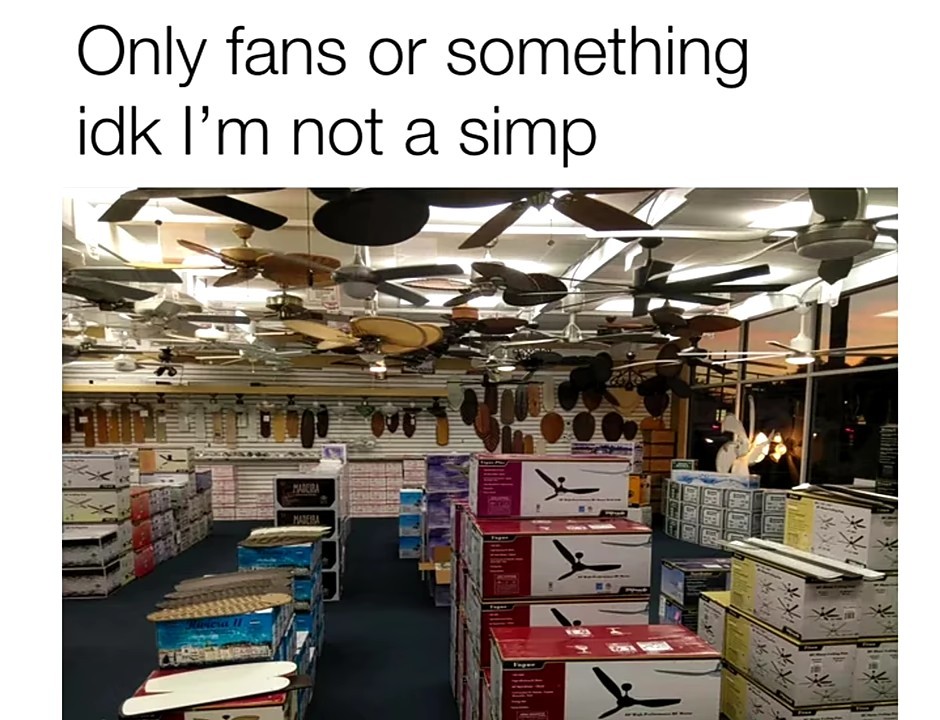In the meme image, a humorous text at the top reads in black on a white background: "Only fans or something, IDK, I'm not a simp." The scene below depicts an indoor retail setting specifically an aisle in a store dedicated to ceiling fans. The store has ceiling fans displayed at the top and shelves filled with various fan boxes in colors like red, blue, yellow, and predominantly white. The boxes are stacked horizontally and there are approximately 20 fans showcased at the top of the image. On the ground, there's a dark blue carpet, and the back wall suggests a display of different ceiling fan blades, colors, and styles. Overall, the store specializes in ceiling fans and related accessories.